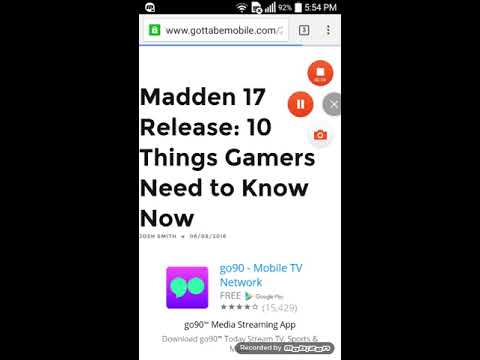The image is a detailed screenshot from an older Android phone display. At the top, the website URL field shows "www.gottabemobile.com" with a green lock symbol next to it, indicating a secure connection. To the right of the URL, a box indicates three tabs are currently open. The device time is shown as 5:54 PM and the battery is at 92%. Below these icons, there is a red-circled pause button, a red-circled stop button above it, and a gray-circled X-out button to the bottom right, indicating the use of a screen recording software displaying icons for pause, stop, and exit. 

The article's headline in the screenshot reads: "Madden 17 Release: 10 Things Gamers Need to Know Now." At the bottom of the screen, there is an advertisement banner for the "Go90-MobileTV Network," which is described as free and available on Google Play, with a 4 out of 5-star rating from 15,429 reviews. The app description includes "Go90 media streaming app download Go90 today stream TV sports" before being cut off. The screen has thick black borders on either side, characteristic of older Android phone screenshots.